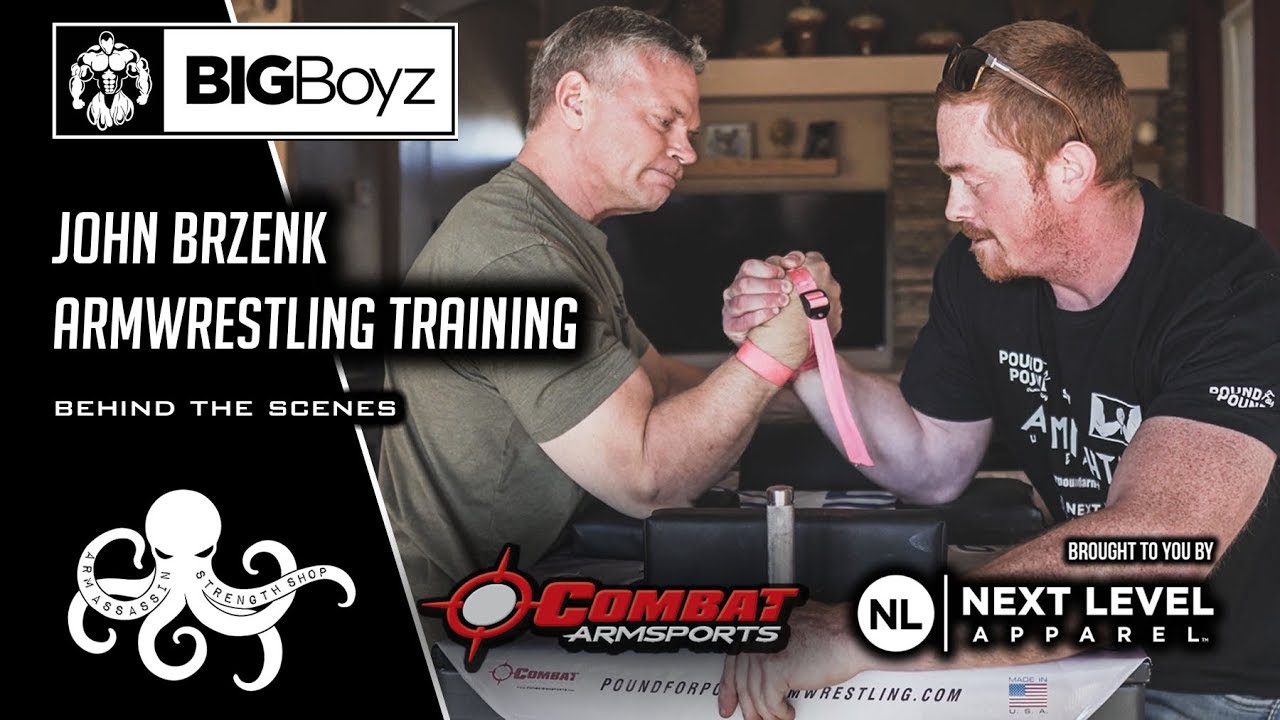This detailed and cohesive caption combines the shared and emphasized details from the three initial descriptions:

This advertisement for Combat Arm Sports prominently features two men engaged in a heated arm-wrestling match. The man on the left, wearing a green short-sleeve shirt, has gray short hair and a grimacing expression, with his bulging biceps straining as he wrestles his opponent. On the right, the man has reddish hair, a short cut, and sports a mustache and goatee, with sunglasses perched on top of his head. He is dressed in a black shirt with indistinguishable writing on it. Their right arms are tightly clasped together and secured with a pink strap, over a mat. 

Above the image, in the top left corner, there is a box featuring a hand-drawn or computer-generated outline of a bodybuilder. Beside this outline, in large letters, it reads "Big Boys." Beneath it, in white lettering, it states "John Brzenk Arm Wrestling Training Behind the Scenes." Below this, there is a logo of a white octopus, with the words "Arm Assassin Strength Shop" written on its tentacles. Along the bottom, in red letters, it says "Combat Arm Sports," and adjacent in white letters, it reads "Brought to You by Next Level Apparel," with a circular logo displaying the initials "NL."